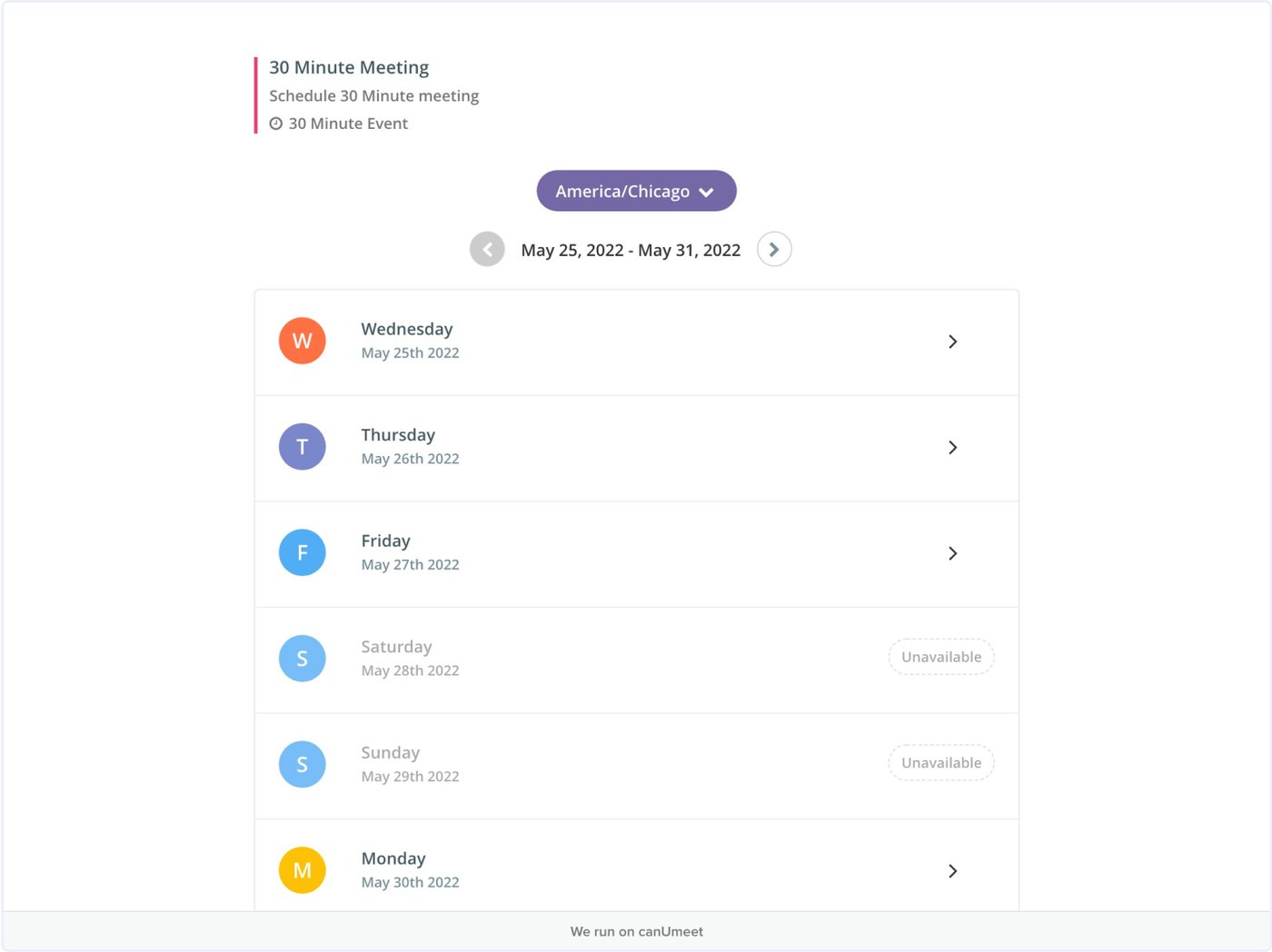The image appears to be a section of a travel website focused on scheduling meetings. In the top left corner, there's a maroon (or violet) line with the text, "30-minute meeting," adjacent to it. Below this heading, it reads, "Schedule 30-minute meeting," accompanied by a clock icon, followed by "30-minute event."

In the central section of the image, there's an oval-shaped button with a purple background displaying "America/Chicago" next to a drop-down arrow. Below this, still centrally located, there is a gray circle with a left-pointing arrow and the text "May 25, 2022 - May 31, 2022" placed in between. Adjacent to this text, there's a white circle with a right-pointing arrow.

The next row lists dates and days of the week starting with "Wednesday, May 25, 2022," followed by "Thursday, May 26, 2022," "Friday, May 27, 2022," each with right-pointing arrows on their right-hand side. Next to these dates are circular icons containing the initial letters of the days. Beneath Friday, the sequence continues with "Saturday," "Sunday," and "Monday," maintaining the same format, except for Saturday and Sunday, which lack the right-pointing arrows.